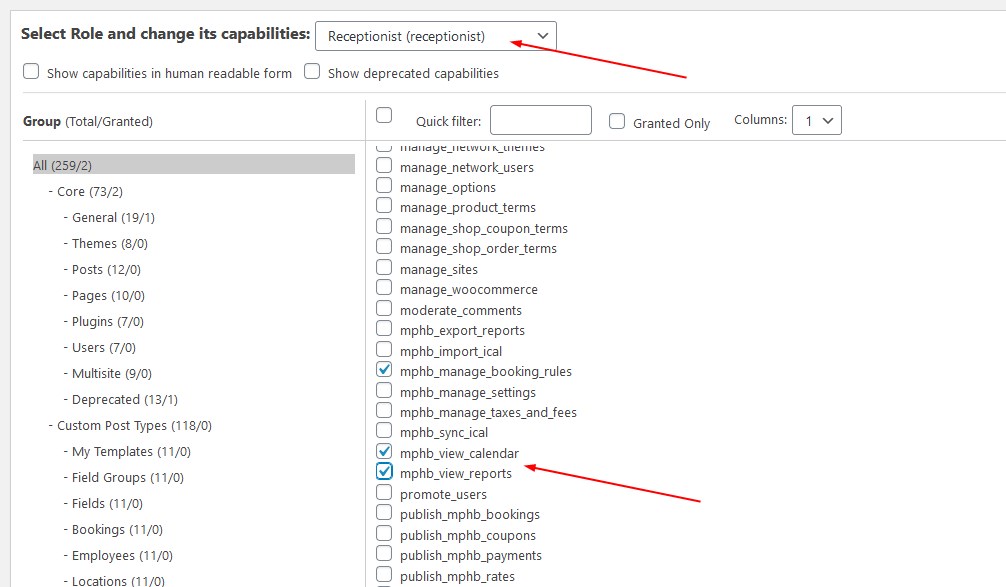This image is a screenshot from a software configuration utility page, likely intended for use by IT professionals. The interface features a clean, white background, and though the names of the software and company are not visible due to the cropped view, several interface elements are clearly identifiable. 

In the upper left corner, bold black text instructs users to "Select Role and Change Its Capabilities." Adjacent to this instruction is a gray-outlined dropdown menu displaying the word "receptionist," repeated in parentheses, with an upside-down triangle indicating the menu can be expanded. A thin red arrow points to the word "receptionist," signifying its importance or selection.

Below this, there are options to customize the viewing of capabilities: "Show capabilities in human readable form," which features a gray checkbox, and "Show deprecated capabilities," allowing further customization. 

On the left side of the page, a section titled "Group (total/granted)" displays a list of items categorized by their functions, including "core," "general," "themes," "posts," "pages," "plugins," "users," "multi-site," and "deprecated." 

To the right of this section is a column with a detailed list of specific capabilities, such as "manage_network_users" and "manage_options." Another red arrow points to an item labeled "MPHB_view_calendar," drawing attention to this specific capability.

This detailed configuration page exemplifies the granular control afforded to IT professionals when managing user roles and their associated capabilities within the software.